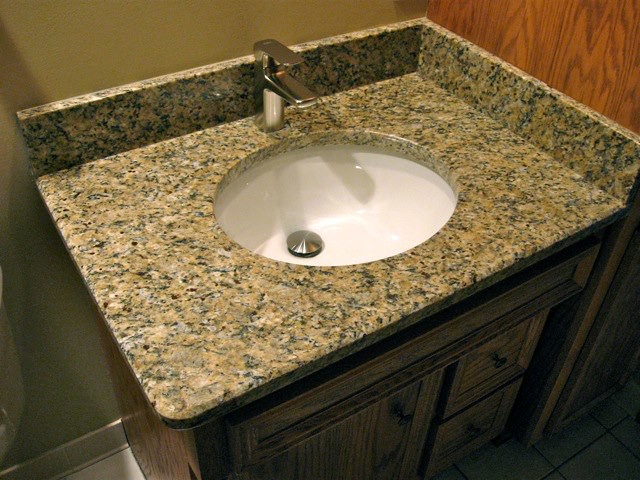A detailed photograph taken inside a bathroom features a dark-finished wood vanity cabinet. The cabinet has a combination of a single door on the left and multiple drawers on the right. Atop the cabinet rests a polished granite countertop with a blend of brown, beige, and black speckles, lending a luxurious touch to the setting. Centrally positioned in the countertop is a round white sink, above which is a modern, single-handled faucet. The walls of the bathroom are painted in a medium pea green color, reminiscent of split pea soup, adding a unique ambiance to the room. To the right of the vanity area, a side view of a medium wood-colored storage cabinet is visible, contributing additional utility to the space. The room is devoid of any text or additional decorative elements, focusing solely on the clean and functional design elements.